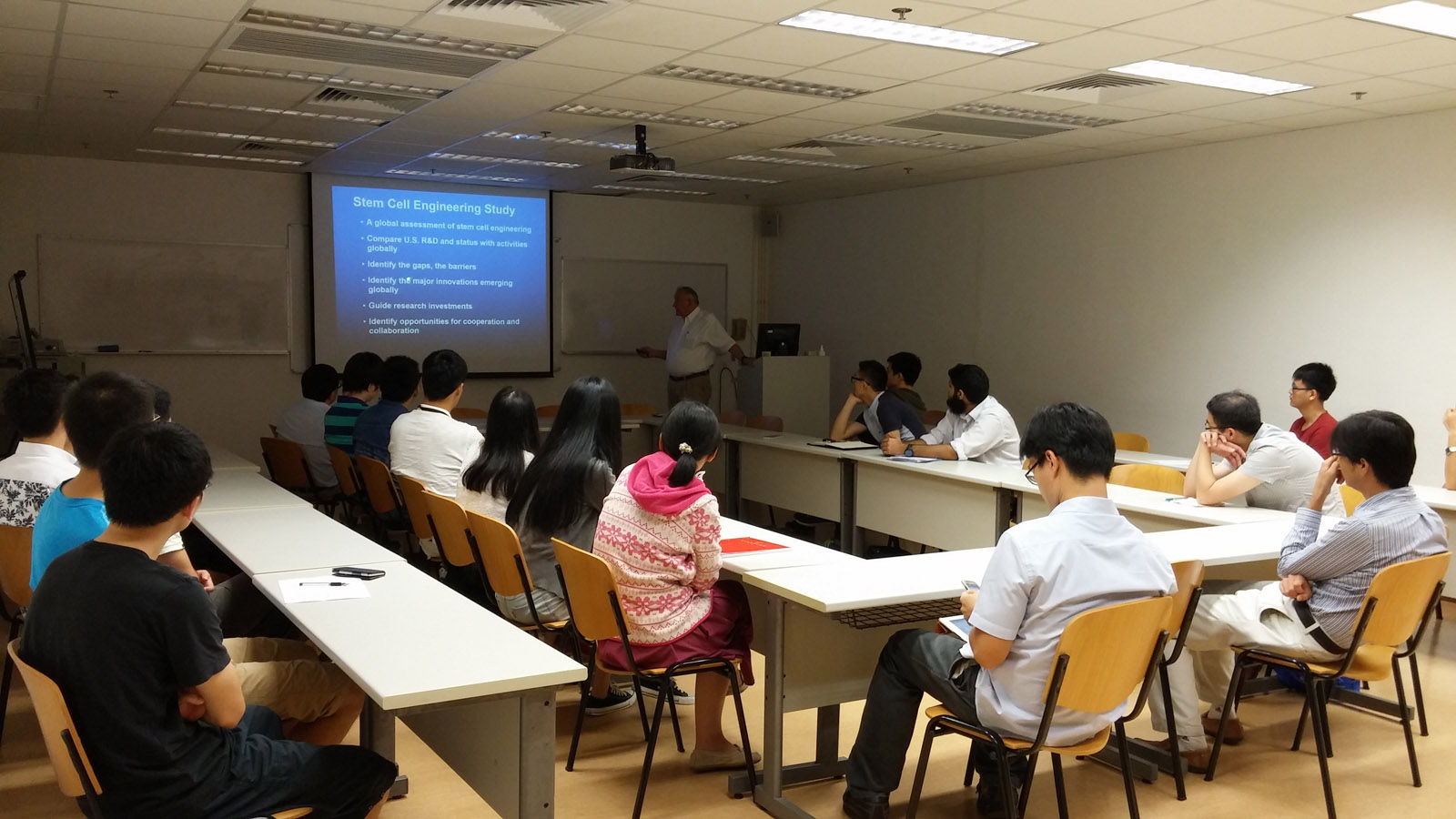The photograph shows a spacious classroom with a modern design. At the far end of the room, a teacher stands beside a large screen displaying a blue projection that reads "STEM Cell Engineering Study." Engaged in his lecture, the teacher faces the class, pointing towards the screen.

On the left side of the image, four desks are grouped together, each with a clean, white rectangular surface. On the right side, desks are arranged in a U-shape, fostering a collaborative learning environment. The students, notable for their dark hair, are attentively focused on the teacher, some with hands resting in their laps, while others have their elbows propped on the desks. 

The classroom is well-lit by fluorescent ceiling lights, interspersed with vents. The back wall is pristine white, adorned with two dry erase boards flanking the projection screen. The wooden chairs, each with a supportive back, match the wooden flooring that adds warmth to the modern educational setting.

Overall, this is a dynamic and interactive STEM class in session, emphasizing collaborative and focused learning.